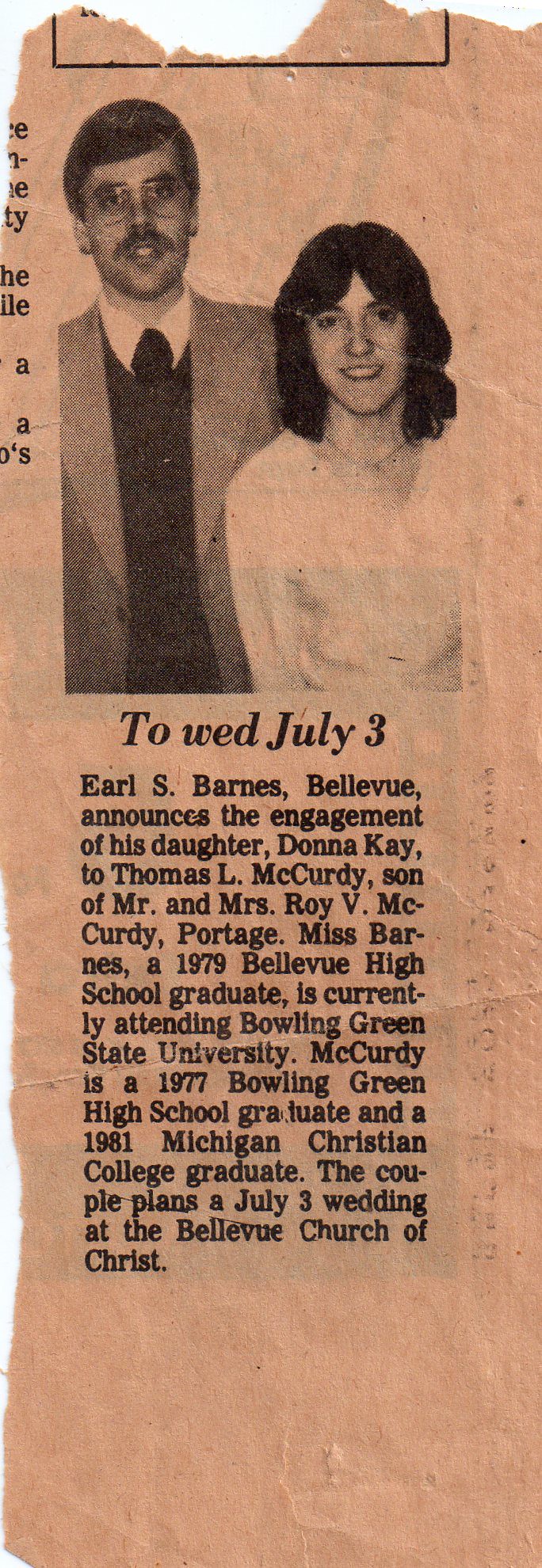The image is a vintage black-and-white newspaper clipping, slightly tinted with pink, announcing the wedding of Donna K. Barnes and Thomas L. McCurdy, set for July 3rd. The top half features a formal portrait of the Caucasian couple, with the man on the left and the woman on the right, both smiling and looking at the viewer. The man, about a head taller than the woman, has light black hair, wears glasses, a gray jacket with a shirt and tie, and sports a dark mustache. The woman has shoulder-length black hair and is dressed in a light-colored or white dress. The announcement text below the photograph reveals that Earl S. Barnes of Bellevue is announcing the engagement of his daughter, Donna K. Barnes—a 1979 Bellevue High School graduate currently attending Bowling Green State University—to Thomas L. McCurdy, the son of Mr. and Mrs. Roy V. McCurdy of Portage. McCurdy is a 1977 Bowling Green High School graduate and a 1981 Michigan Christian College graduate. The couple plans to wed at the Bellevue Church of Christ. The layout is typical of a single-column newspaper announcement, combining detailed text with black-and-white imagery.